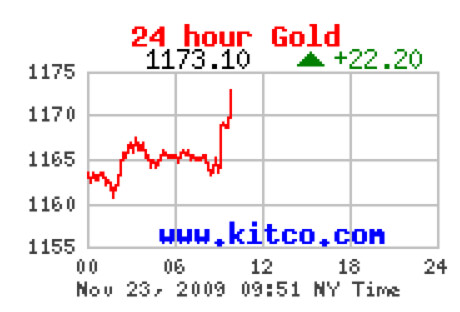The image is a screenshot of an old, basic graphical chart from November 23, 2009, at 9:51 AM New York time, sourced from kitco.com. Dominating the image is a 24-hour gold price chart, denoted by the red text "24-hour Gold" at the top. The current price of gold is prominently displayed in black text as 1173.10, accompanied by a green up-arrow indicating a price increase of 22.20. The chart tracks gold prices ranging from 1155 to 1175, with time markers at 00, 06, 12, 18, and 24 hours along the bottom. The price fluctuations are depicted by a red line moving across the chart. The provider's website, kitco.com, is visible at the bottom, confirming the source of the stock ticker chart.